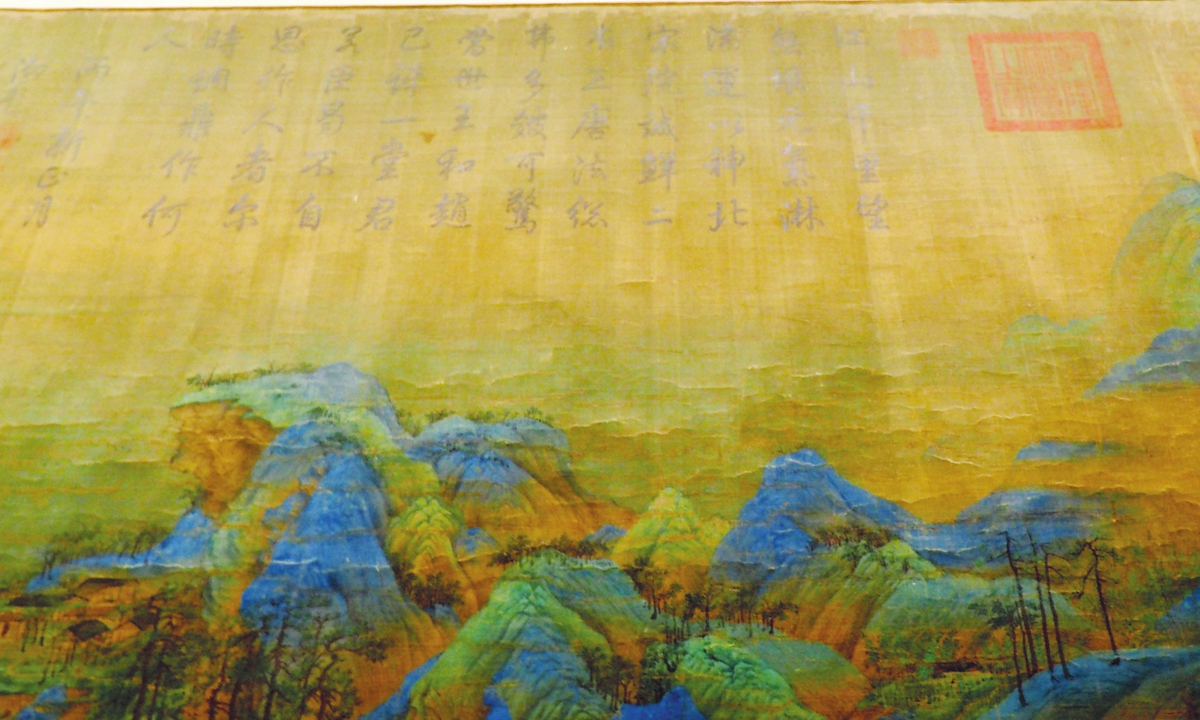This is a vintage landscape painting, likely created on aged paper or cloth, displaying a distinctly cracked texture indicative of its age. The painting predominantly features an autumn scene with a rough landscape, including both mountains and trees in an array of blue, green, gold, and brown hues. At the top, a cascade of Chinese characters written in black runs across the yellowed background, accompanied by a red stamp or square symbol in the upper right corner. The mountains, which shift in color from blue at their peaks to green and yellow towards their bases, are dotted with scattered, sparse trees. In the bottom left corner of the painting, four small buildings appear to be elevated from the ground. The sky above the mountains is depicted in shades of green, adding a unique touch to the overall composition.